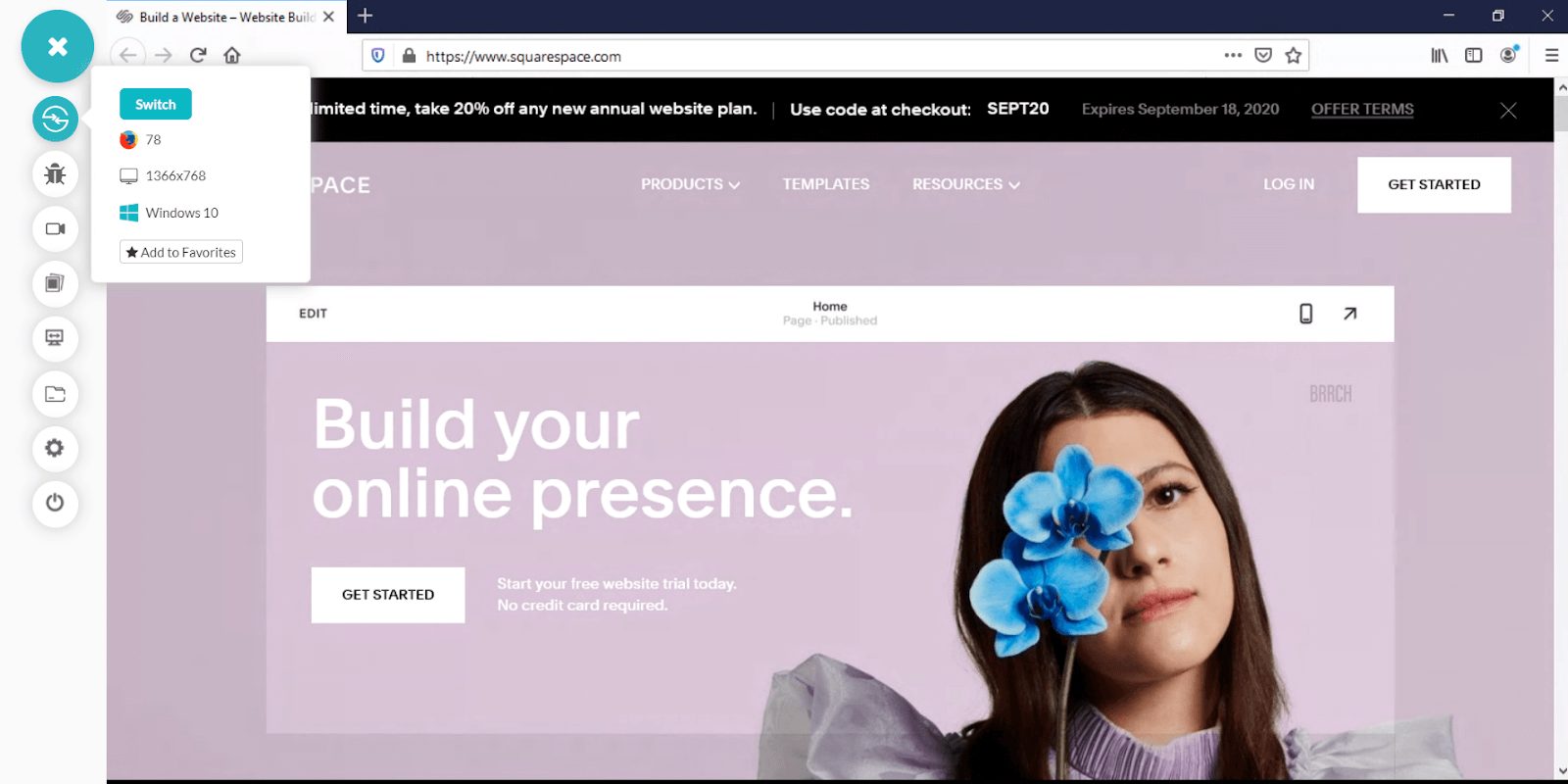The image is a rectangular screenshot from a website, with the longer sides being the top and bottom. On the left edge of the screenshot, there is a light gray vertical banner running from the top to the bottom. Along this banner, there are several circular icons representing different user options or settings.

At the top of the banner is a large green circle with a white 'X' symbol. Below it, there is a smaller green circle featuring a white circle with a line through its center; to the right of this icon, a white rectangular pop-up menu appears with the text "Switch." 

Adjacent to the pop-up menu, the familiar Firefox browser logo, a fox encircling a globe, is visible. Next to this logo, the numeral '78' is displayed. Following this, the dimensions "1366 x 768" are listed alongside a monitor icon. Nearby, the Windows logo appears with the text "Windows 10" next to it, and a black text rectangle stating "Add to Favorites."

Returning to the sidebar, the next icon is a white circle depicting a bug, indicating a troubleshooting or bug reporting option. Below this, a white circle displays a camera icon, likely for capturing screenshots. Following this is another white circle with two overlapping photographs, hinting at a gallery or media manager.

Further down, there is a white circle with a square containing two lines, possibly representing a document or a textbox. Directly below this is the outline of a file folder within a white circle, indicating file management. The next icon is a white circle containing a cogwheel, typically representing settings. The final circle at the bottom contains the power symbol, a circle with a dash at the top, likely for logging out or shutting down.